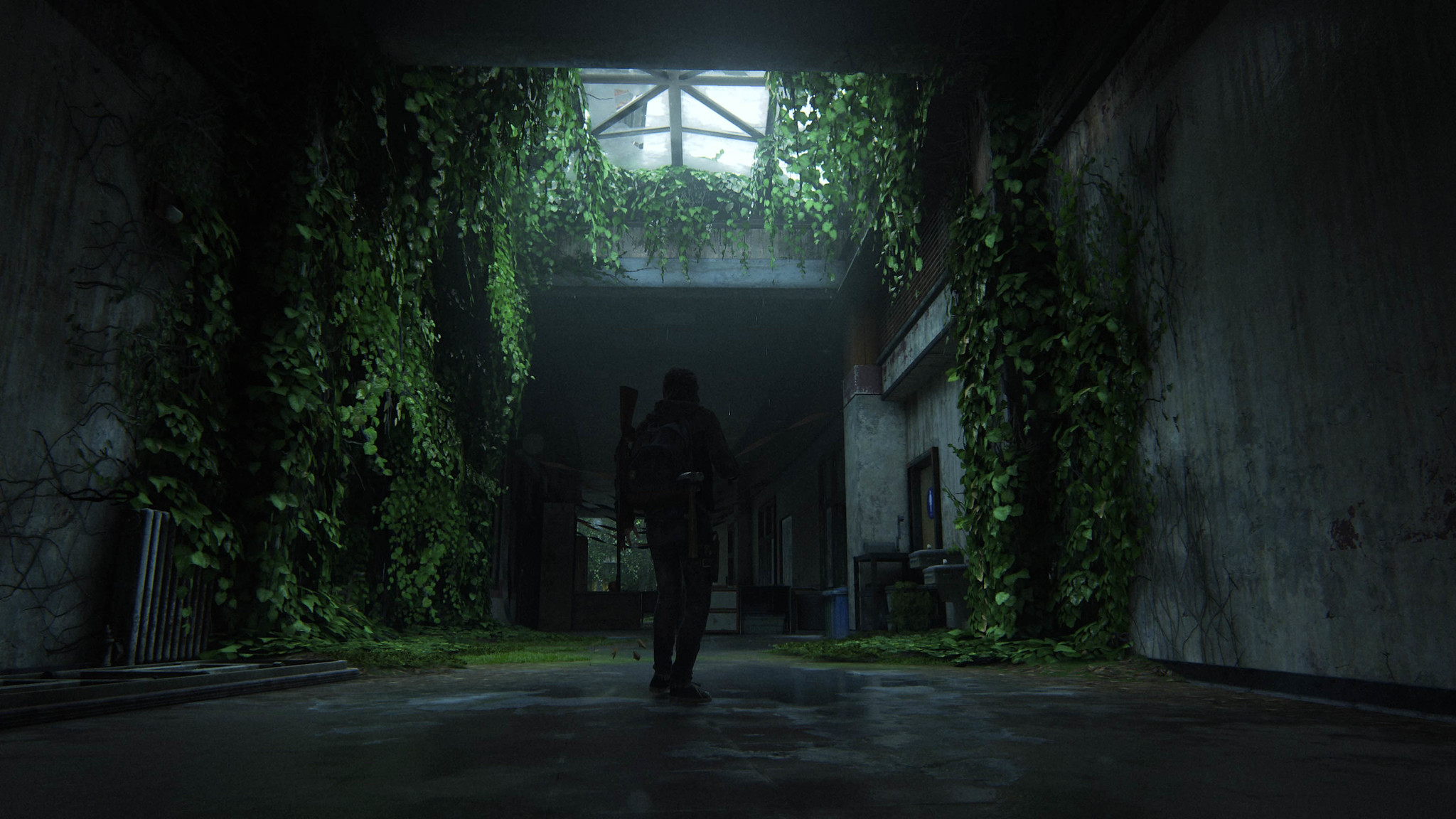A captivating interior scene reveals a blend of nature and architecture. The right wall is constructed from gray stone, giving the space a rugged and timeless appearance. The floor is also made of stone, but patches of grass have taken root, adding a layer of green to the room. Vines climb the left wall, adorned with an abundance of green leaves that cascade down and stretch across the ceiling. At the bottom left corner, a radiator peeks out amidst the lush greenery. 

The skylight above lets in a touch of daylight, mingled with icy patterns, hinting at a cold environment outside. From the ceiling, more vines and leaves hang down, creating a canopy of foliage that frames the scene. The right side of the image also features a dense collection of green leaves, adding to the room's verdant ambiance.

At the center of this overgrown yet enclosed space, a lone figure stands, holding a pistol grip rifle in their left hand. Their posture suggests they are alert and on guard, locked into this untamed, yet architecturally intriguing building.